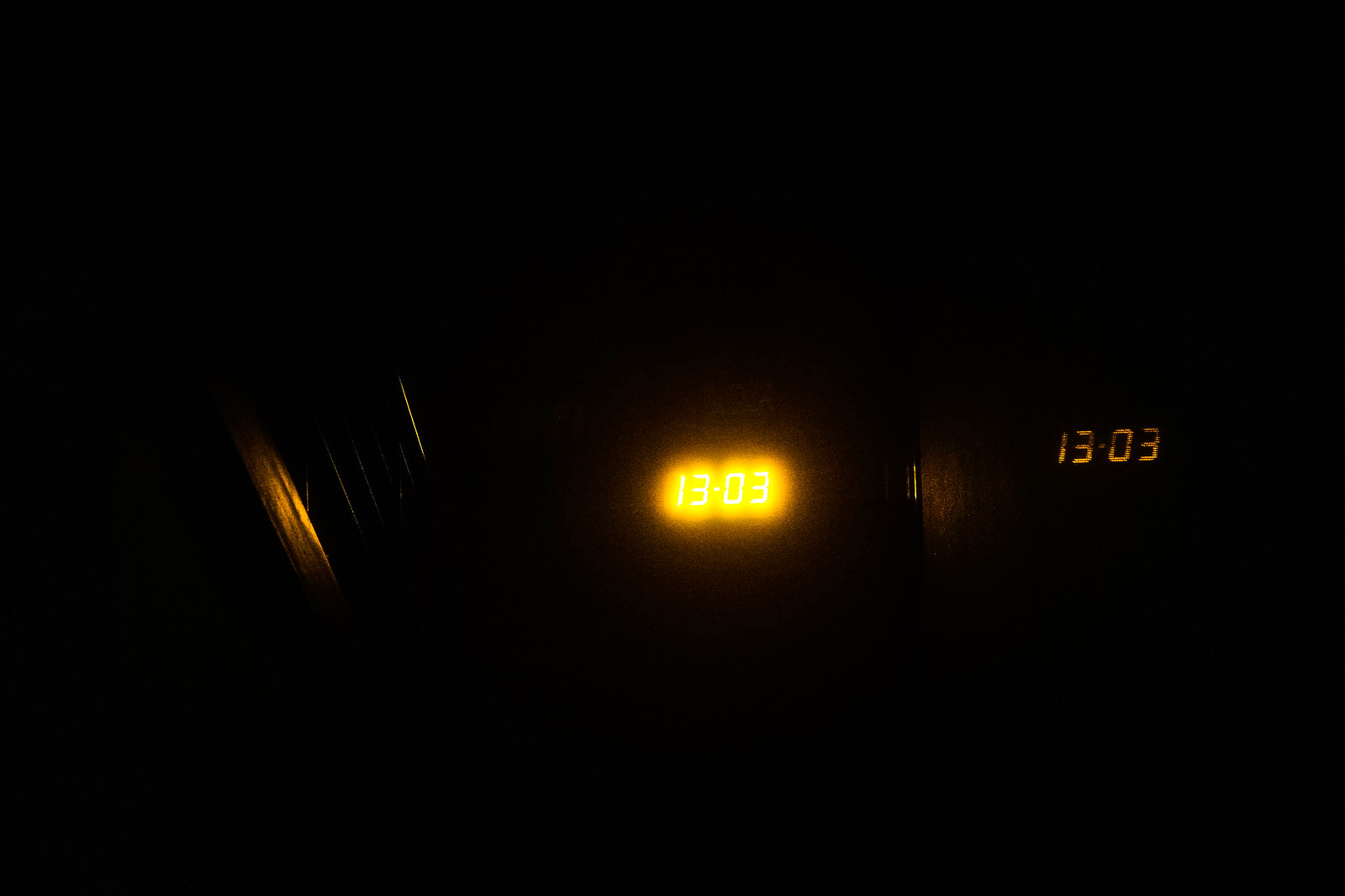The image is predominantly dark, with only a few discernible elements illuminated in the middle while the rest is shrouded in pitch black. At the center, there is a vibrant, bright yellow clock face displaying '1303' in white digits. This clock is encircled by a warm red-orange glow, making it the primary light source in the image. To the right of this clock, another clock face, also showing '1303', appears but lacks the surrounding glow, characterized instead by lit-up numerals that don’t illuminate the surroundings. On the left side of the image, an indistinct object is faintly visible, illuminated by the glow emanating from the brightly lit central clock.